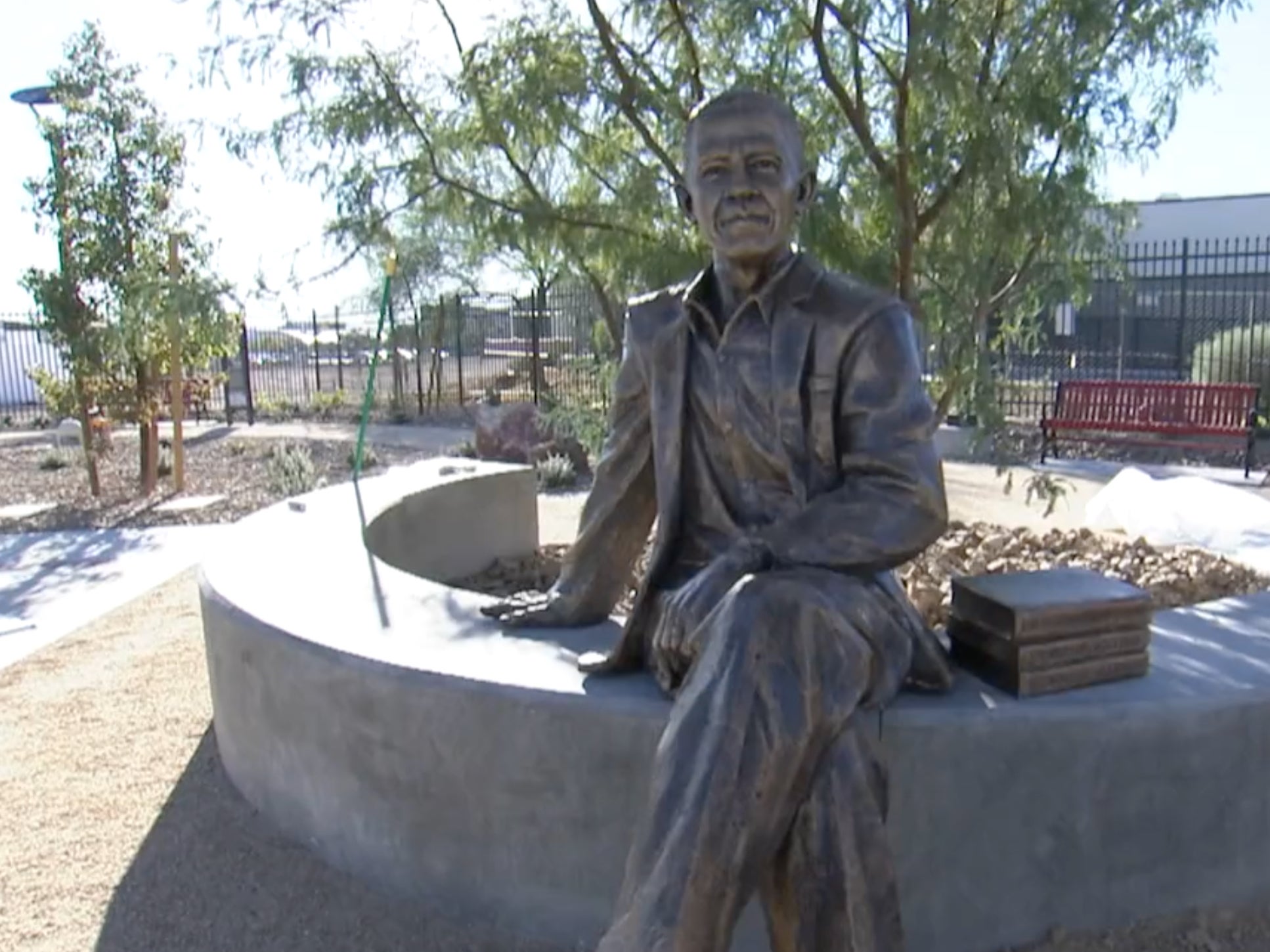The photograph depicts a serene community park with a central focus on a detailed, greyish metal statue of a seated man. The statue, appearing proud and contemplative, is dressed in a jacket, button-down shirt, and pants, with one arm resting over his leg and the other placed on his lap. Beside him are three sculpted metal books. He is seated on a concrete half-circle ledge. The park setting includes a variety of greenery, with trees scattered throughout and a large tree with lush green leaves directly behind the statue. In the background, there are benches – one is brown with black legs, while another is noted as red – and a black metal fence that encloses the area. The pathways weave through the verdant space, creating an inviting, tranquil atmosphere, and the high fence, possibly about eight feet tall, suggests the park is designed to keep visitors, especially children, safely inside.